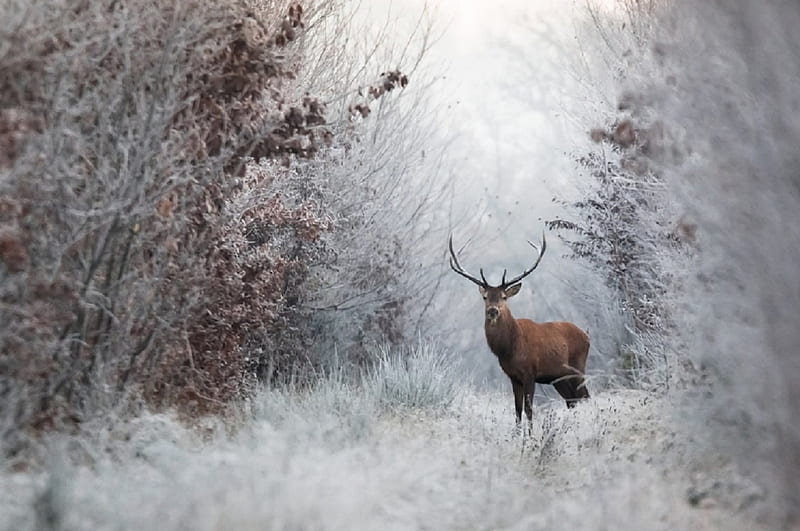In this photograph, a muscular, brown deer with prominent antlers stands in the center of a foggy, winter forest. The scene on both the left and right of the image is dominated by trees, some adorned with brown and red leaves, indicative of the fall season, while others are bare. A light dusting of snow, inferred from the whitish hues on the trees and the tall, unmown grass below, hints at an early winter setting. The fog intensifies towards the center of the image, creating a slightly out-of-focus effect on the foreground and right side, while the area to the left remains more defined. The deer, facing slightly to the left but looking straight ahead, is perfectly poised with its symmetrical antlers extending upwards in several points, creating an almost surreal, ethereal quality to the scene. The overall smoothness of the image and the silky texture of the deer's fur evoke an otherworldly, almost AI-generated feel to the photograph.